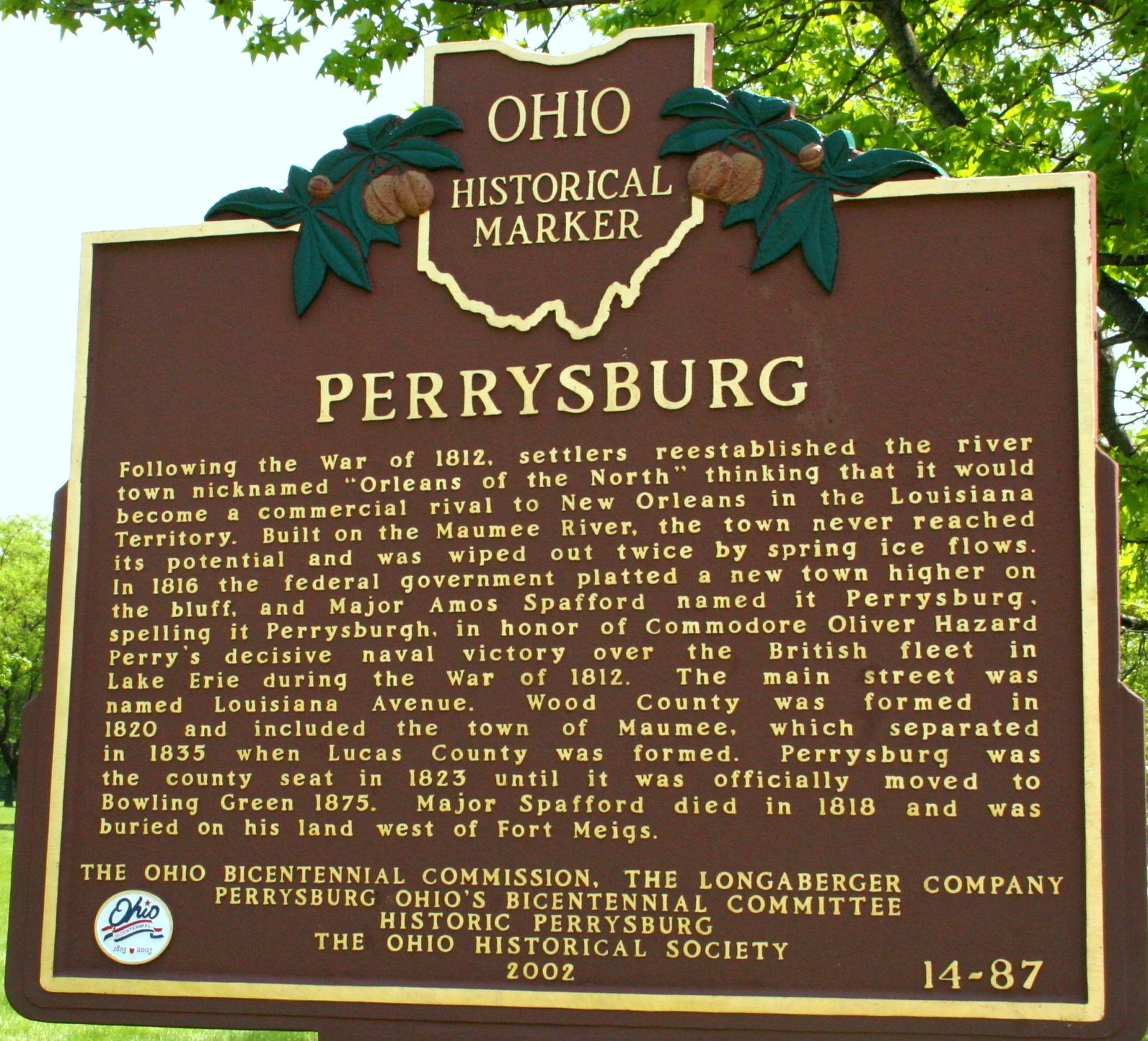This photograph captures a prominent historical marker from Ohio, titled "Perrysburg." The marker, supported by a post and set against the backdrop of a lush, mid-summer tree with green leaves, predominantly fills the frame. Crafted in an almost square, brown design, the plaque features the Ohio Historical Marker emblem at the top, displaying a map of Ohio flanked by small decorative elements resembling acorns or coffee beans.

The detailed inscription on the marker recounts the post-War of 1812 history, where settlers reestablished a river town named Orleans of the North along the Maumee River. Originally envisioned to rival New Orleans commercially, the town was devastated twice by spring ice flows. In 1816, the federal government platted a new town on higher ground, naming it Perrysburg, after Commodore Oliver Hazard Perry, who triumphed over the British fleet in Lake Erie. This new town featured Louisiana Avenue as its main street. Perrysburg served as the county seat of Wood County from 1823 until 1875, when it was moved to Bowling Green. Major Amos Spafford, who named Perrysburg, died in 1818 and was buried west of Fort Meigs.

The marker was installed in 2002 by multiple organizations, including the Ohio Bicentennial Commission, the Longaberger Company, Perrysburg, Ohio's Bicentennial Committee, Historic Perrysburg, and the Ohio Historical Society, identified as marker 14-87.